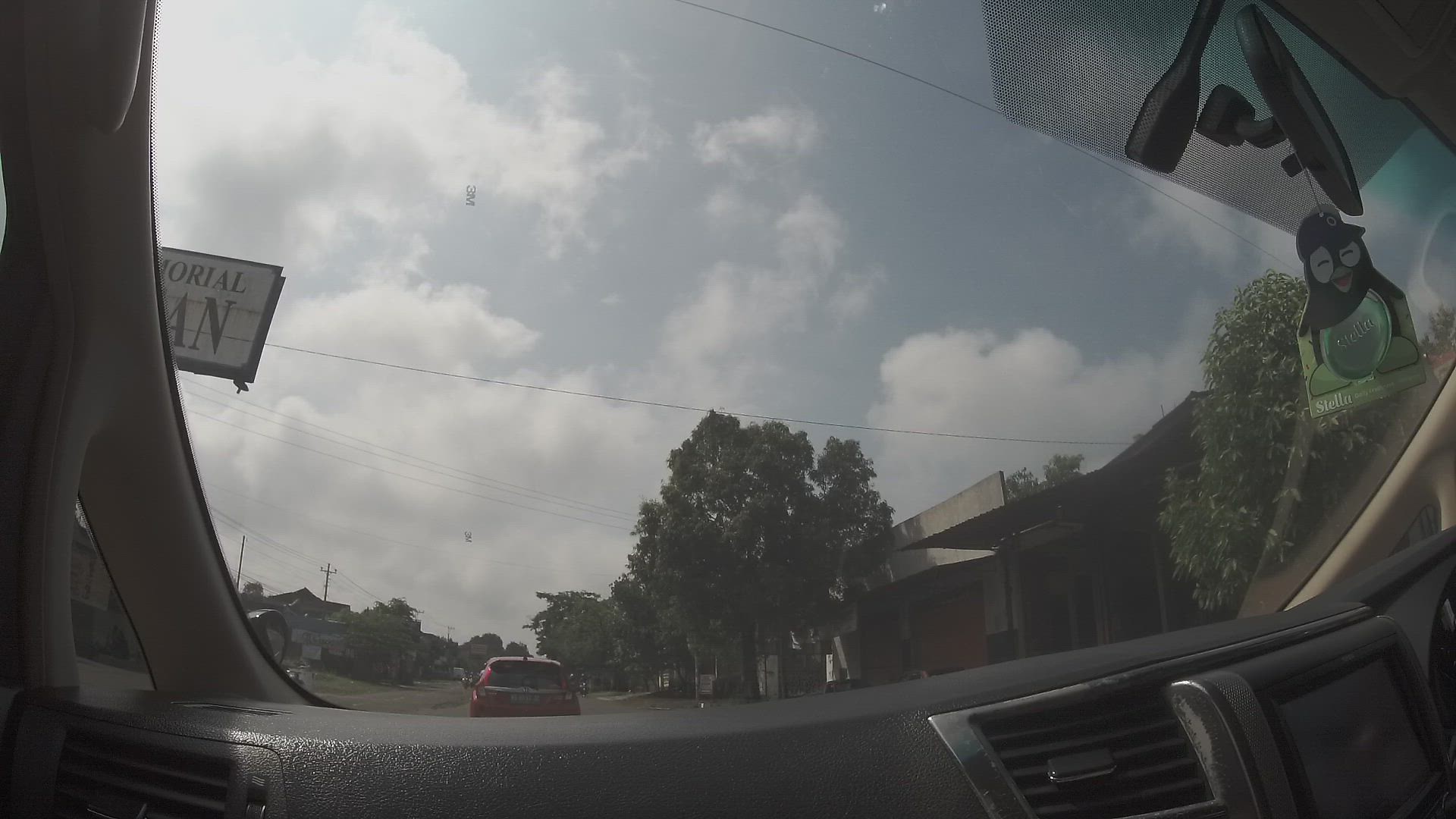A wide-angle shot taken from inside a car, showcasing the entire front windshield. The image appears slightly stretched, enhancing its panoramic effect. At the center of the rearview mirror hangs a penguin-shaped air freshener, adding a whimsical touch. The weather is sunny, with a vibrant blue sky speckled with a few white clouds. Outside, a serene residential neighborhood is visible, characterized by lush green trees, bushes, and an array of homes. The car is parked on the right-hand curb of the road, while a red car is stationed in front of it. The street is also dotted with garages, adding to the suburban ambiance.